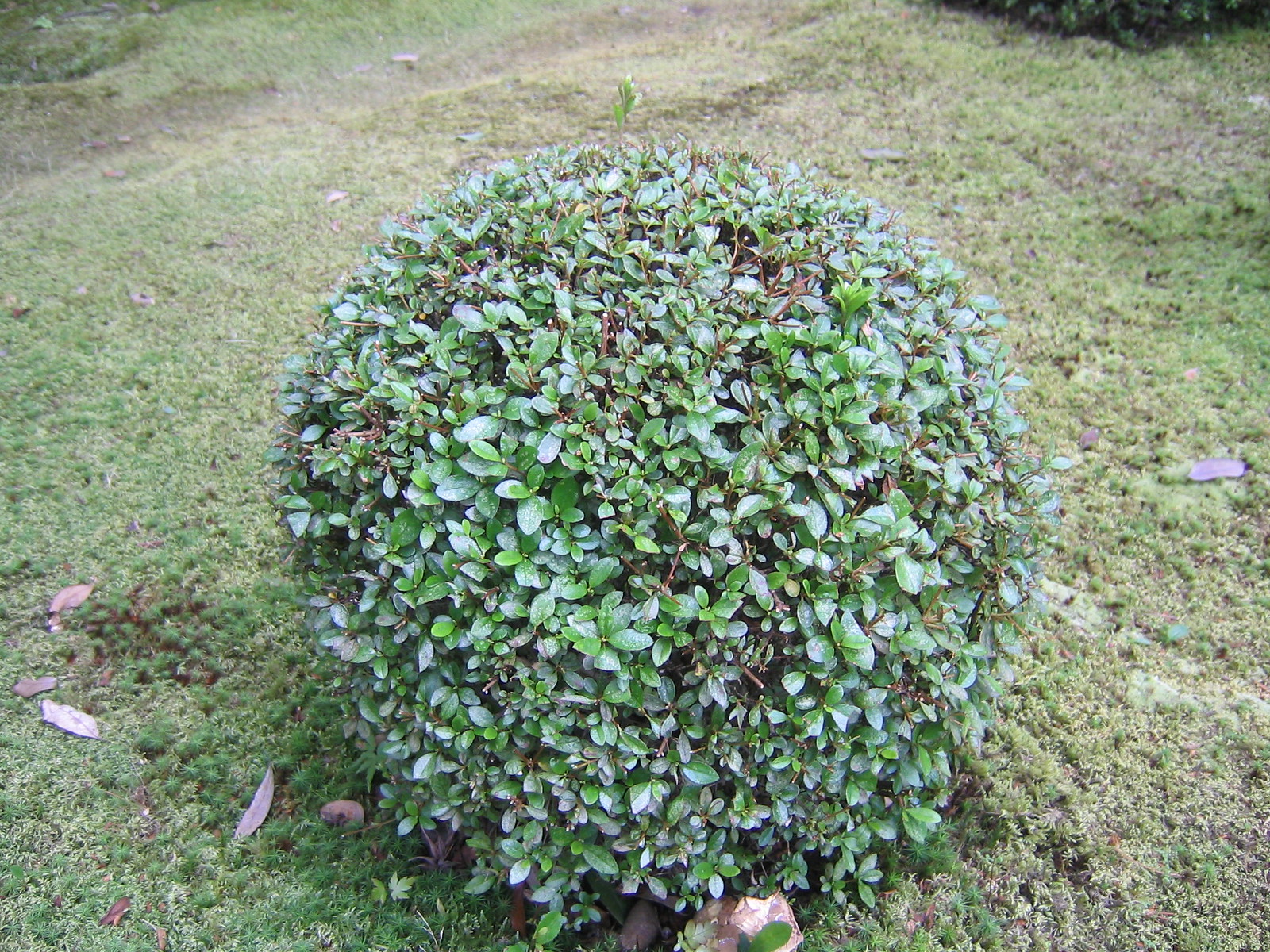This image features a meticulously manicured, perfectly spherical bush set in the middle of a grassy field. The close-up reveals a variety of leaf sizes, grouping together in a manner reminiscent of flower petals. The surrounding grass is predominantly green, though patches of yellow and brown suggest areas of dying grass. The ground is sparsely populated with debris, including some dried leaves and what look like brown feathers. A noticeable amount of dirt is visible through the short grass. A solitary rock or similar object is partially tucked under the bush in the foreground. No other bushes or trees populate the immediate vicinity, with the exception of one additional bush visible in the upper right-hand corner of the image. The scene, devoid of text, presents a calm landscape characterized by various shades of green, brown, and black.